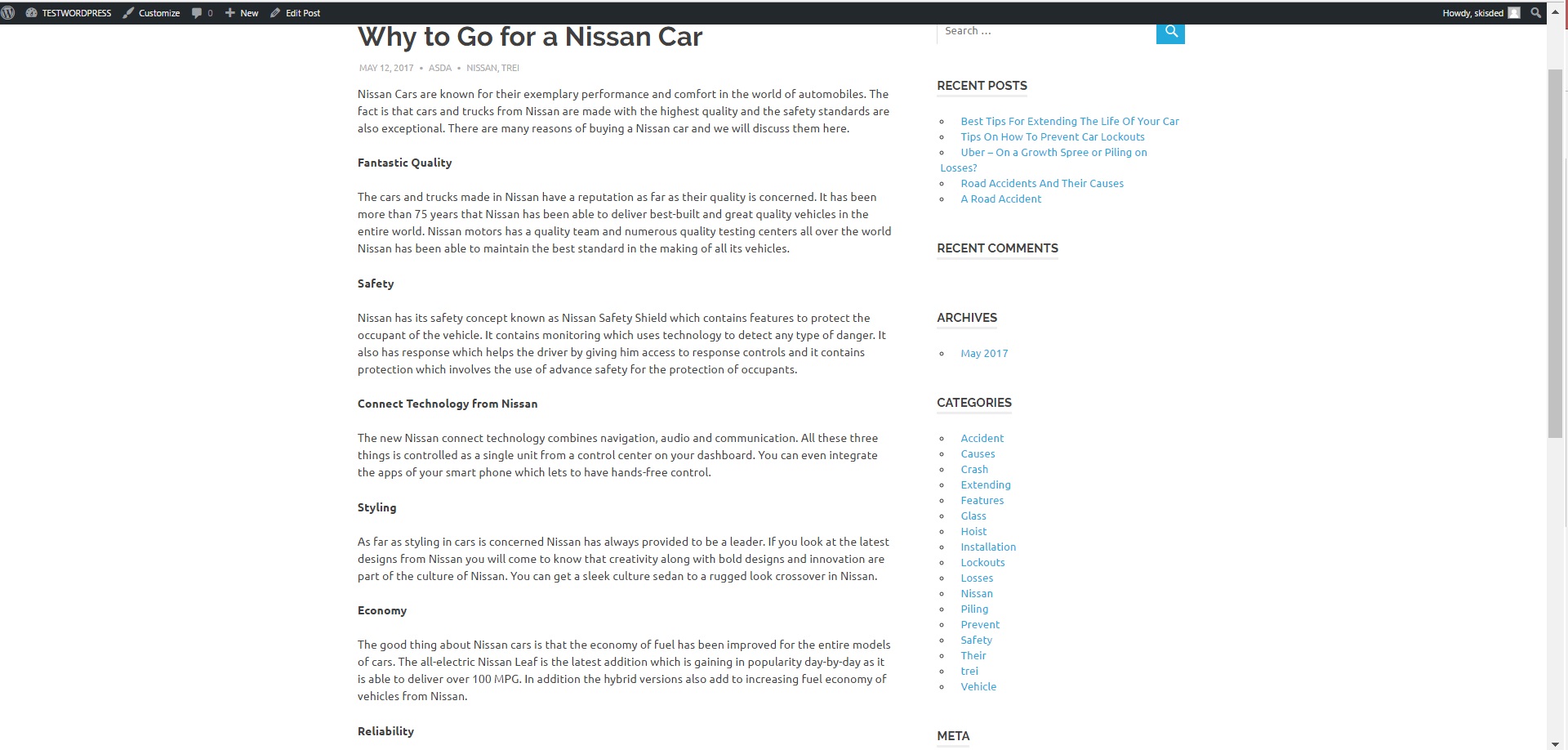The image appears to be a screenshot of a website or an app, its width roughly 50% to nearly 100% greater than its height. At the top, there's a thin black bar stretching from left to right with some unreadable text on both the upper left and upper right corners.

Below, the main content starts after an indentation of approximately 25-30%. The large title, rendered in black text, reads: "Why Go for a Nissan Car." Following the title is a paragraph and various sections, each introduced by bold black headers. The headers include:

- "Fantastic Quality" with an accompanying paragraph
- "Safety" accompanied by a paragraph
- "Connect Technology from Nissan" followed by a paragraph
- "Styling" with a paragraph
- "Economy" and an associated paragraph
- "Reliability," but the image cuts off before showing its paragraph.

On the right side of the image, there appears to be a sidebar with different sections. The first section, "Recent Posts," lists five distinct links. Below it is the "Recent Comments" section, which currently has no entries. Further down, the "Archives" section lists an entry for May 2017. Following that is a "Categories" section, listing approximately 15 different categories. At the bottom of the sidebar, the word "Meta" is featured.